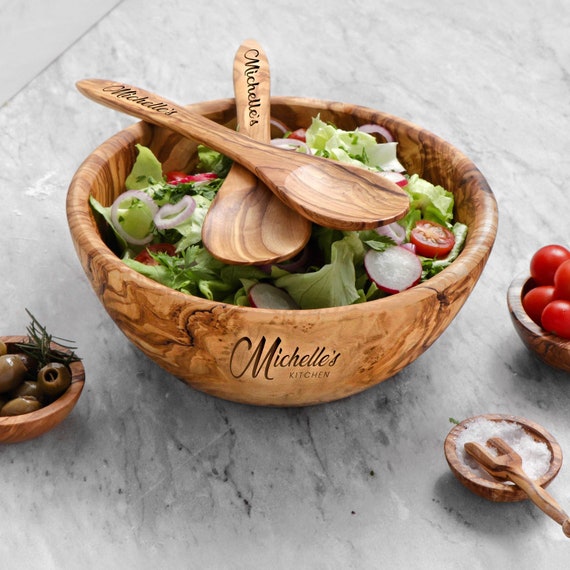The image displays a detailed and vibrant food scene set on a grey ceramic table, characterized by darker black lines or dots. At the center of the table is a large, round wooden salad bowl engraved with the name "Michelle's Kitchen." This bowl is filled with a fresh mix of green lettuce, cherry tomatoes, sliced red radishes, and chopped green and purple onions. Atop the salad, two wooden spoons engraved with "Michelle's" are neatly crossed.

To the left of the salad bowl, there is a smaller, round wooden bowl filled with brown olives. On the right side, a similar wooden bowl contains coarse white salt, and just above it, another small bowl holds more cherry tomatoes. All the wooden bowls and utensils create a harmonious aesthetic against the contrasting grey surface of the table, enhancing the rustic and inviting atmosphere of the scene.